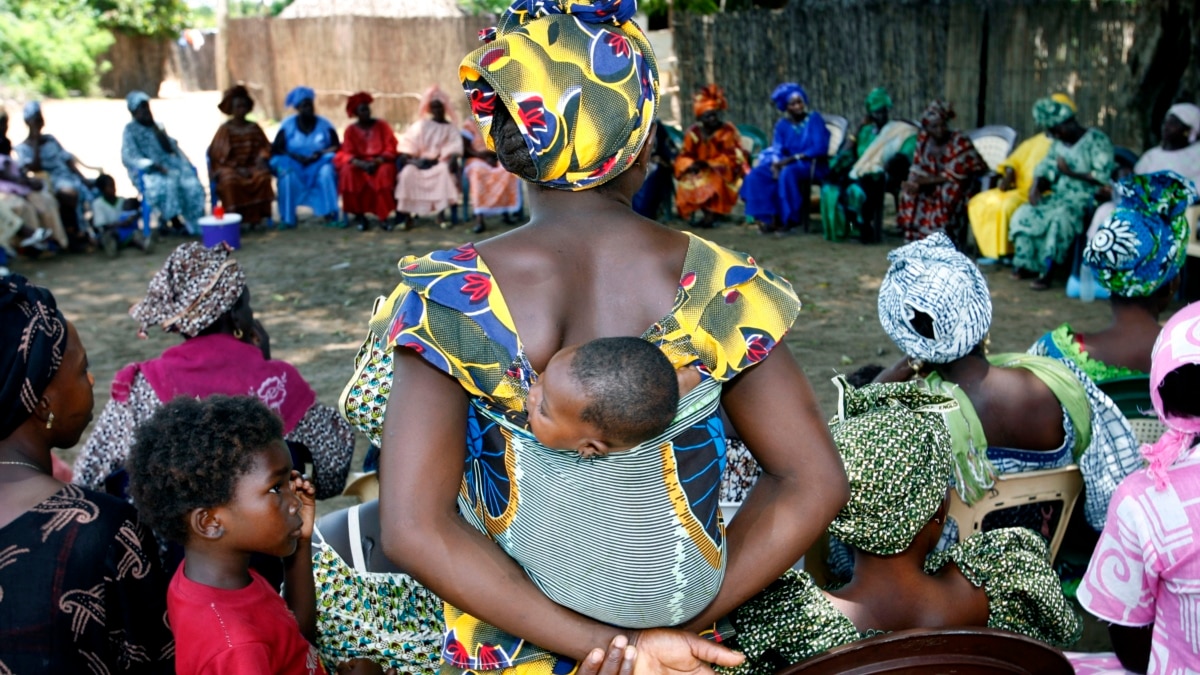The image depicts a vibrant outdoor gathering in an African village, where a diverse group of men, women, and children are seated in a large circular formation on a dirt ground. The villagers are adorned in colorful, pastel-hued robes and billowy hats, reflecting traditional African attire. Central to the foreground is a woman with her back to the viewer, dressed in a unique sleeveless robe, carrying an infant in a sling on her back. The infant's head peeks curiously between the woman's shoulder blades. Nearby, a small child in a bright red t-shirt stands looking towards another part of the circle. Surrounding the gathering is a wooden fence, and green branches and leaves can be seen in the top left corner, adding a touch of nature to the scene. An empty chair and another seated woman can also be noticed among the participants, capturing a moment of communal interaction and cultural richness.